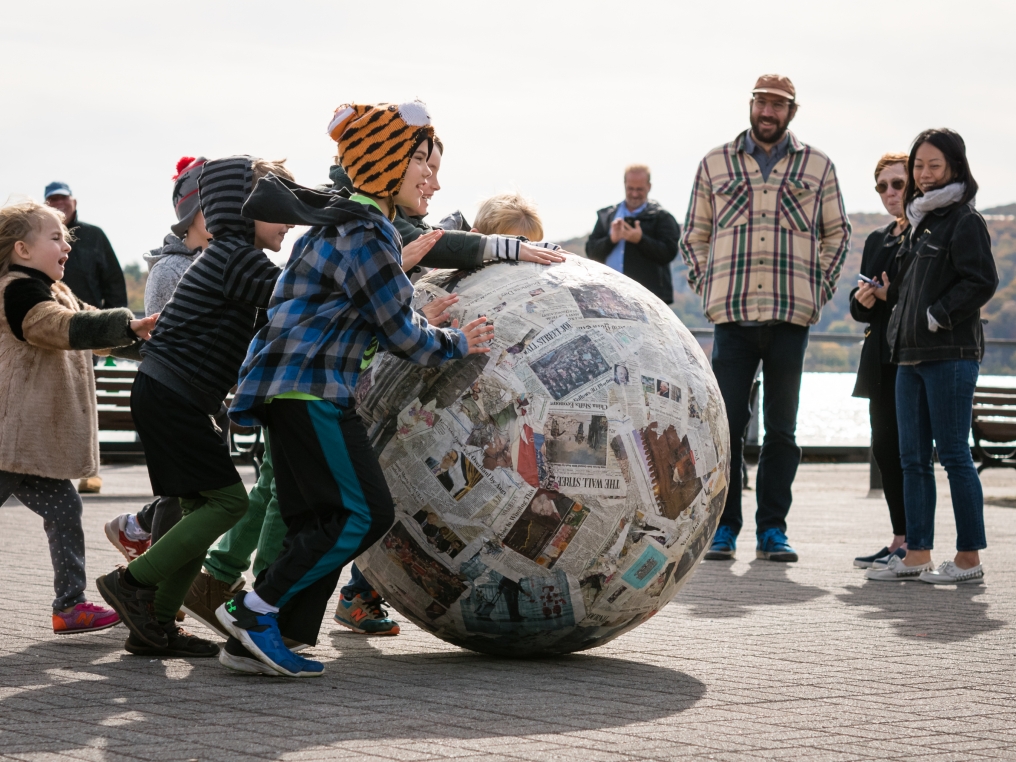In this vibrant photograph, a group of children, dressed in casual clothing and colorful stocking caps, are energetically rolling a massive ball covered in newspaper clippings, stamps, and articles, akin to a papier-mâché creation. The ball, almost chin-high to the children, appears deceptively lightweight as they push it effortlessly. The children, approximately 8 to 9 years old, include mostly boys, with one small girl trailing behind, seemingly trying to catch up to join the fun. In the foreground, a child is notably clad in a blue plaid shirt, dark joggers with a blue stripe, blue shoes, and an orange hat, while another child sports a black and gray hoodie, black shorts, and jeans underneath.

Behind them, a few adults, possibly parents, are watching with smiles, some engaged with their phones, capturing the joyous moment. Among them, an Asian woman and a tall white man in a tan plaid shirt, tan hat, black jeans, and blue sneakers stand out. The background showcases rolling hills or valleys, a body of water, and dark benches scattered around the grey ground, all under an overcast sky, hinting at a cool, yet cheerful day outdoors. The entire scene exudes a sense of community, playfulness, and shared happiness.